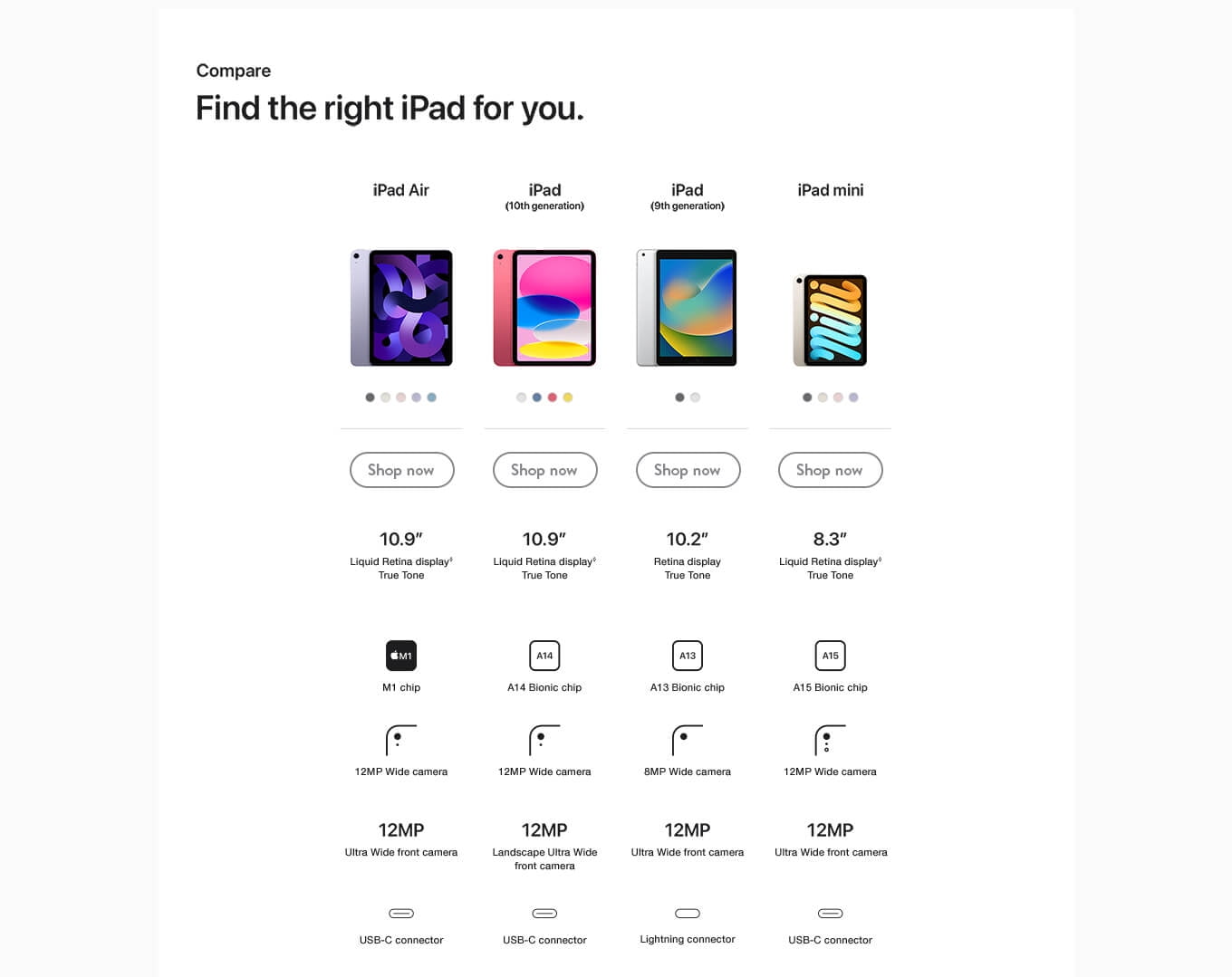This is an informational page designed to compare different iPad models side by side against a white background. Across the top, bold black text reads, "Compare. Find the right iPad for you." Below this headline, four iPad models are listed horizontally in black text: iPad Air, iPad 10th generation (with "10th generation" in parentheses under the designation), iPad 9th generation, and iPad mini. Each iPad is depicted with a full-color screen image beneath its respective name.

Under these images, there are rows of colored dots indicating additional comparison options. Below these rows, a white, oval-shaped button labeled "Shop Now" in gray text invites further action. Beneath this button, detailed information about each iPad is provided, including screen sizes varying from 10.9 inches down to 8.3 inches. Additional specs such as 12 MP camera specifications, battery life, and Bionic chip types are also listed to help inform the buyer's decision.